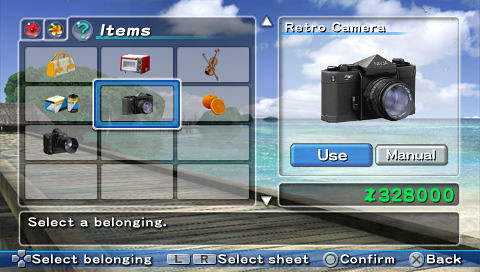The image is a screenshot from a video game interface, featuring a wider-than-tall aspect ratio. The background depicts a serene beach scene with blue skies, clouds, blue water, and a wooden walkway. The left-hand side of the screen displays a semi-transparent grid titled "Items," consisting of 12 options arranged in 3 columns and 4 rows, showcasing various items like a handbag, a violin, a purse, a box, an orange, a larger camera, and prominently, a camera in the center box, which is highlighted. At the bottom, there are navigation prompts including "Select a belonging," "LR," "Select sheet," "Confirm," and "Back."

On the right-hand side, there is a larger, white square box containing a detailed image of an old DSLR camera labeled "Retro Camera." Below the camera image are two buttons: one labeled "Use" on the left and another labeled "Manual" on the right. Beneath these buttons, the number "328000" is displayed in light green. This section also features text instructing "Select a belonging."